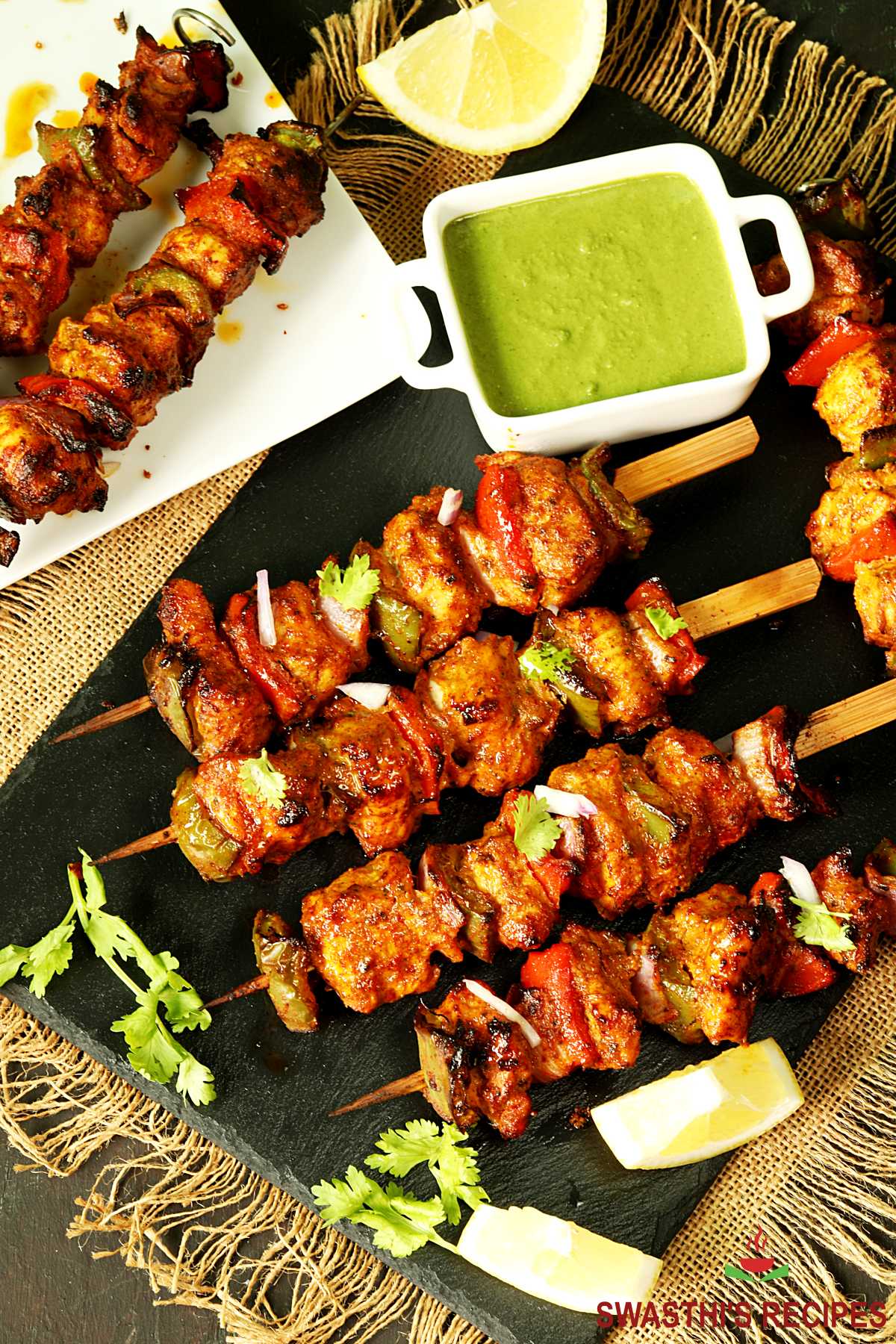This photograph showcases a meticulously arranged meal featuring skewers of meat and vegetables. The rectangular image centers on a black tray set atop a tan, fringe-edged burlap placemat. The primary focus is on five skewers aligned diagonally, each alternating between chunks of meat, red bell peppers, and possibly onions or a white vegetable. Adding to the visual appeal are sprigs of parsley scattered around and lemon slices placed strategically. A notable element is a small, shallow white dish with tiny handles, filled with green sauce, located on the tray. In the top left corner of the image, part of a white plate with two additional skewers is visible. The scene is anchored by atmospheric elements of the placemat and tray, complemented by a logo and text at the bottom right corner, indicating "Swasthi's Recipes."